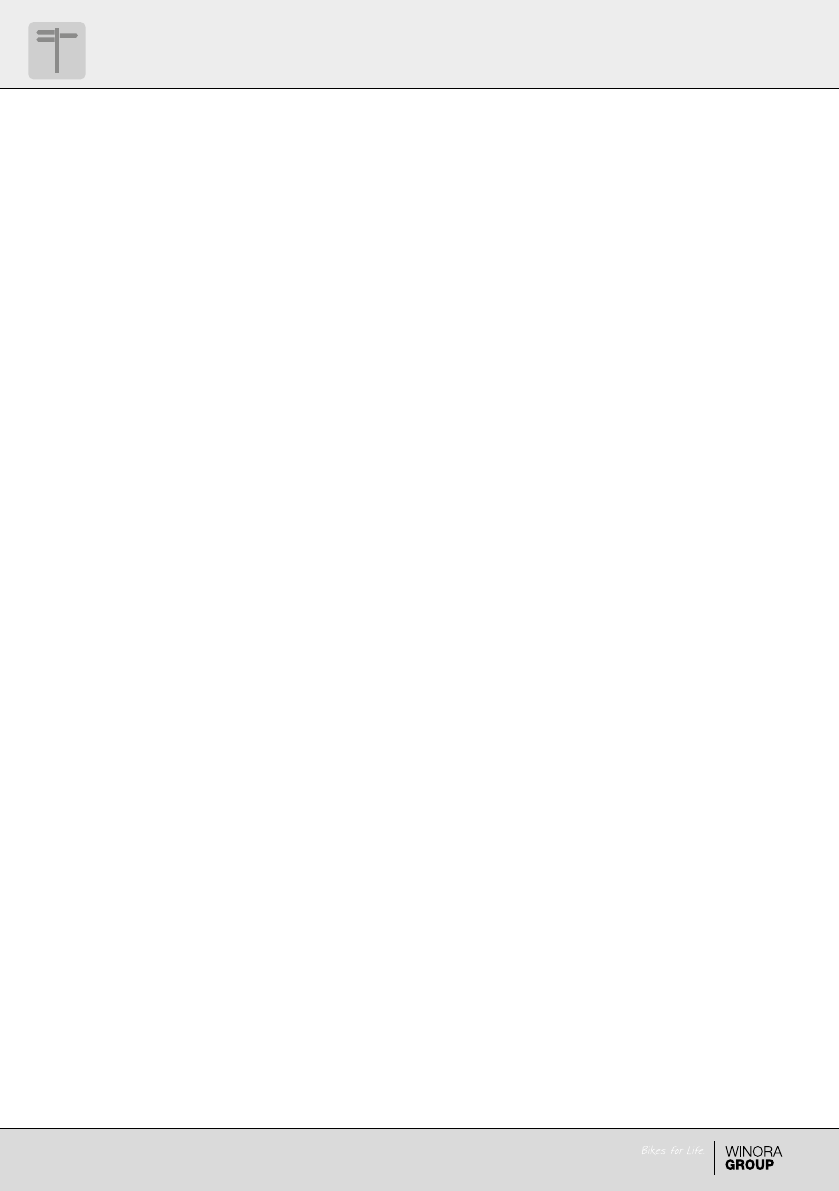This image is a minimalistic and somewhat simplistic long screenshot, structured into three distinct horizontal sections, each with a different background color. The uppermost and bottom rows both feature a gray background and are bordered by a black underline.

In the top-left corner of the first row, a dark gray square is present. Within the square, there appears to be an icon resembling a telephone pole or flagpole, consisting of a vertical line with two horizontal lines extending to the left and one to the right. This row concludes with a simple underline in black, running the entire length of the row.

The central section of the image is a large white rectangle that dominates the screenshot. This area is blank with no text or graphical elements, suggesting an empty state or a placeholder.

In the bottommost row, the gray background continues with a black stripe running horizontally within it. Positioned toward the right-hand corner of this row, the italicized text "Bikes for Life" can be seen in white. Following this, there's a black stripe, and next to it, the text "Winora Group" appears, with "Winora" in regular font and "Group" in bold.

The overall impression of the screenshot indicates a potential display of a webpage that is not fully loaded or is devoid of content, signifying that it might not be functioning correctly.